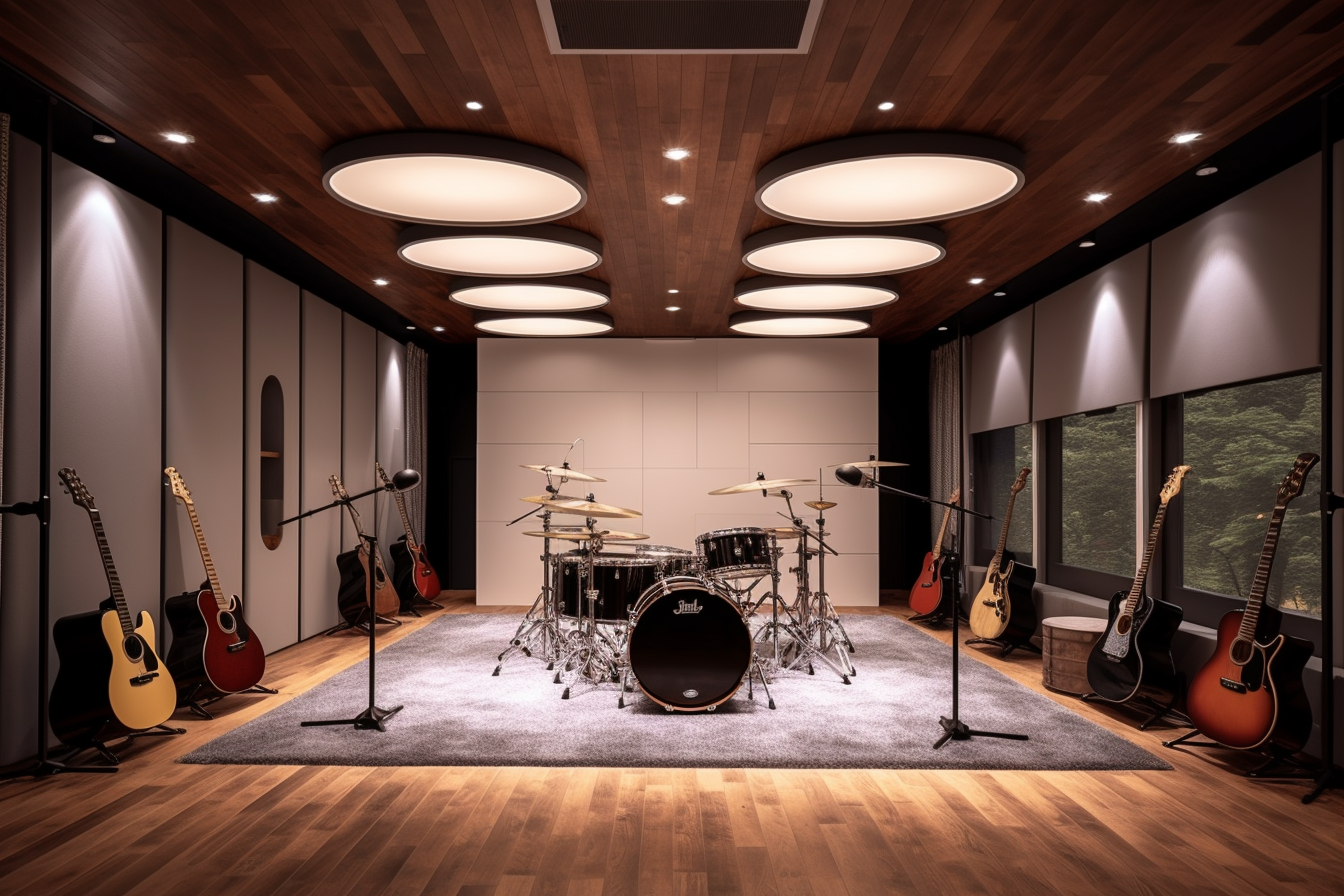The image depicts a modern music studio, characterized by its perfectly rectangular shape and a blend of contemporary design elements. The room features a dark brown, wooden, paneled ceiling adorned with eight large, round drop lights, complemented by recessed lighting. The walls alternate between white or gray panels, and the right side is lined with three large windows covered with white shades, showcasing a view of pine trees outside.

The studio floor is light brown wood, predominantly covered by a gray carpet, especially in the center where a black drum set with multiple cymbals is placed. Surrounding the perimeter of the room are different wood-grain acoustic guitars, with four carefully arranged on each side of the space. Two microphone stands are positioned centrally, enhancing the studio's utility for music production. The overall aesthetic is clean and modern, with the white, well-lit background contributing to the airy and open feel of the space.